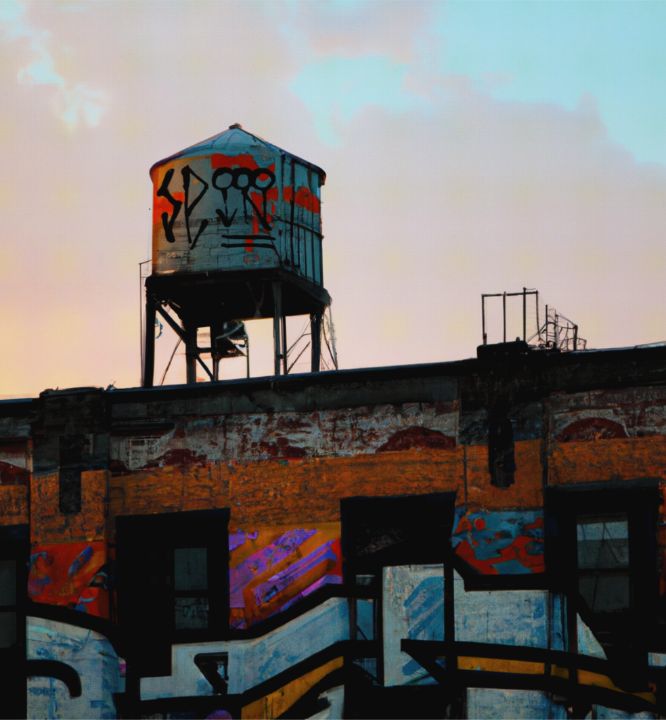In this close-up urban photograph, an old brick building and a small, silo-shaped water tower dominate the scene, both extensively covered in graffiti. The sky, transitioning from a pinkish hue to a soft blue, suggests the image was captured during either sunrise or sunset. The water tower, perched atop the building, features prominent black letters "SP," possibly spelling "SPIN" in ornate detail, alongside symbol-like designs resemblant of the male and female icons. The building itself, possibly abandoned, is adorned with vivid and artistic graffiti in shades of orange, black, off-white, red, gray, blue, and purple. A distinctive tangerine-colored horizontal stripe runs across the brick facade, adding a geometric pattern to the urban canvas. The mix of colors and intricate designs enhances the gritty, artistic atmosphere of this urban landscape.